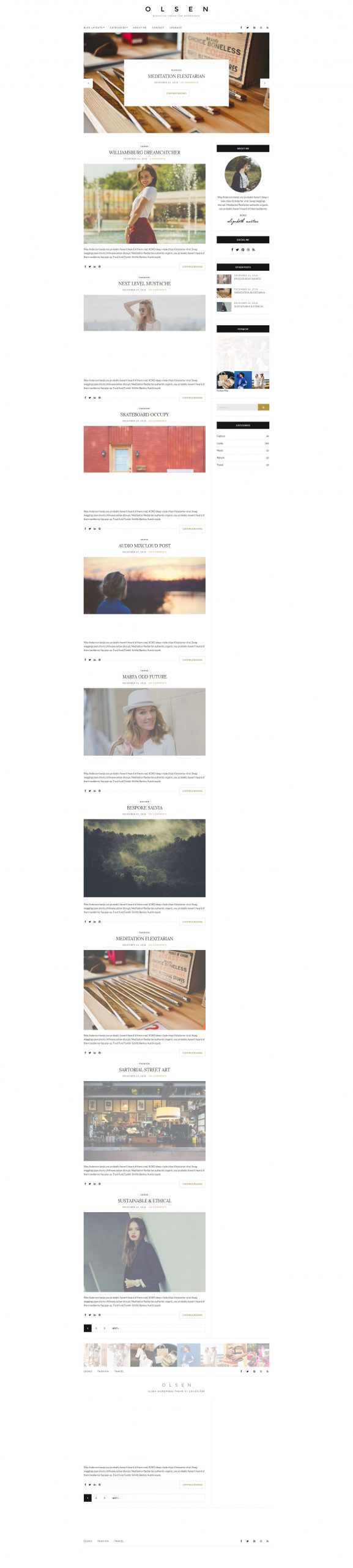A detailed and cleaned-up caption for the image described:

---
The photograph captures a shopping window displayed on what appears to be a PC or a laptop, given the large screen size. The image is sizable, but the details remain minuscule even when zoomed in. At the very top, "Olson" is prominently displayed in darker gray letters against a white background. Below this, there are several text areas on the left-hand side positioned above a rectangular image with five indistinguishable headings. 

A banner graphic, reminiscent of a backgammon table with a white rectangle overlay, features navigation arrows on the left and right. The text on this graphic possibly reads "meditation" or "mediation" in gray lettering.

Continuing downward against a white backdrop, an array of photos is displayed. First, there's an image of a woman in a red skirt and white blouse, seen in profile; this figure is notably blurry. Directly below her, a gray-bannered section shows a woman with long blonde hair and sunglasses, dressed in a white top, with her right arm bent and her hand touching her head, as she gazes to the left.

Next, there is a red wall with a door. Following this, an image depicts the back of an individual in a blue shirt with short blonde hair, standing near what seems to be a bog, lake, or creek. Another photo shows a young woman in a white shirt and white hat, with shoulder-length blonde hair.

Further down, a gray, green, and black image captures the summits of mountains shrouded in stormy clouds and fog. This is followed by the backgammon-style graphic previously mentioned. Two additional photos appear beneath this graphic: one of a storefront and another of a woman dressed in black, likely modeling an outfit. 

At the bottom of the display, a banner features a strip of individual images, each too small to discern.
---